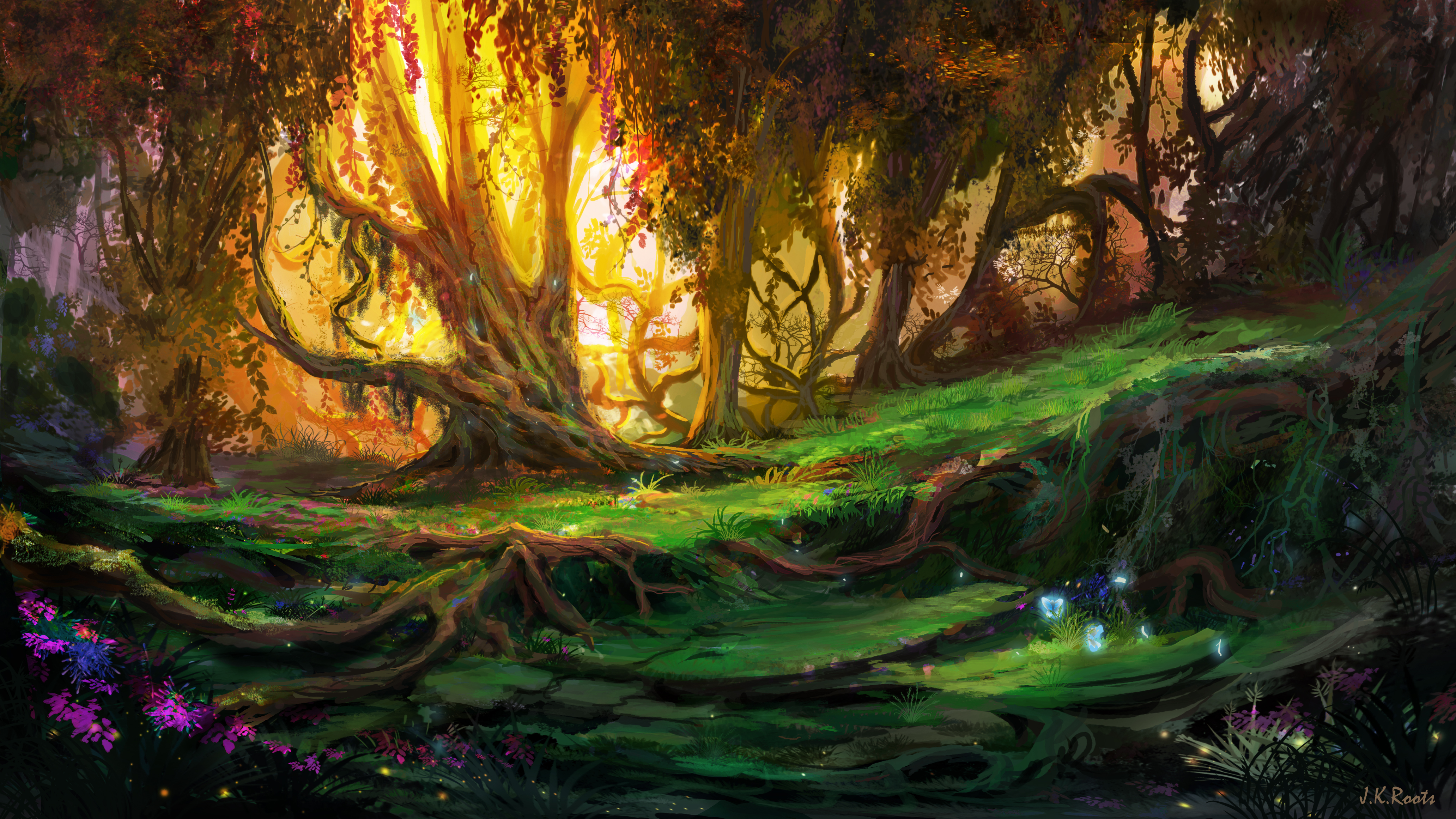This digital painting by J.K. Roots presents a dreamy, fairytale-like forest scene bathed in golden sunlight. The light filters through the gnarled, towering trees in the background, creating a magical atmosphere. The largest tree, positioned in the left third of the image, splits into multiple trunks near its base and is vividly illuminated, drawing the viewer's eye. As the trees recede into the background, they become darker, enhancing the depth of the forest. The lush green ground is crisscrossed with roots and dotted with bright blue and purple flowers, glowing as if lit from within. Fireflies float whimsically around the lower edge, adding to the enchantment. The detailed, smooth painting style contributes to the fantastical feel, rounding out this captivating piece. A subtle watermark in the bottom right corner confirms the artist's identity.